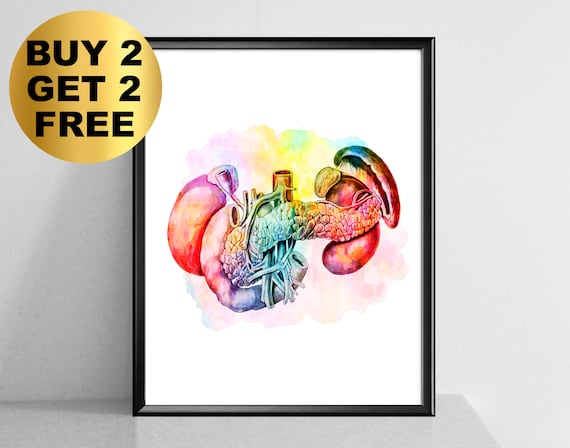This is an advertisement for paintings featuring a striking image of a black-framed poster. In the upper left corner, a large gold circle with black lettering announces a compelling offer: "Buy Two Get Two Free." The central image, set against a completely white background, is a vibrant, multicolored illustration of internal organs including the heart, lungs, liver, and spine. Rendered in watercolor-like washes of reds, yellows, purples, pinks, and blues, the organs are depicted with a mix of anatomical precision and artistic flair. The heart, prominently placed, has visible veins with colorful wisps and overlays that give it a cloud-like, ethereal appearance. The poster is encased in a sleek, skinny, and shiny black frame, adding a polished touch to the overall presentation.